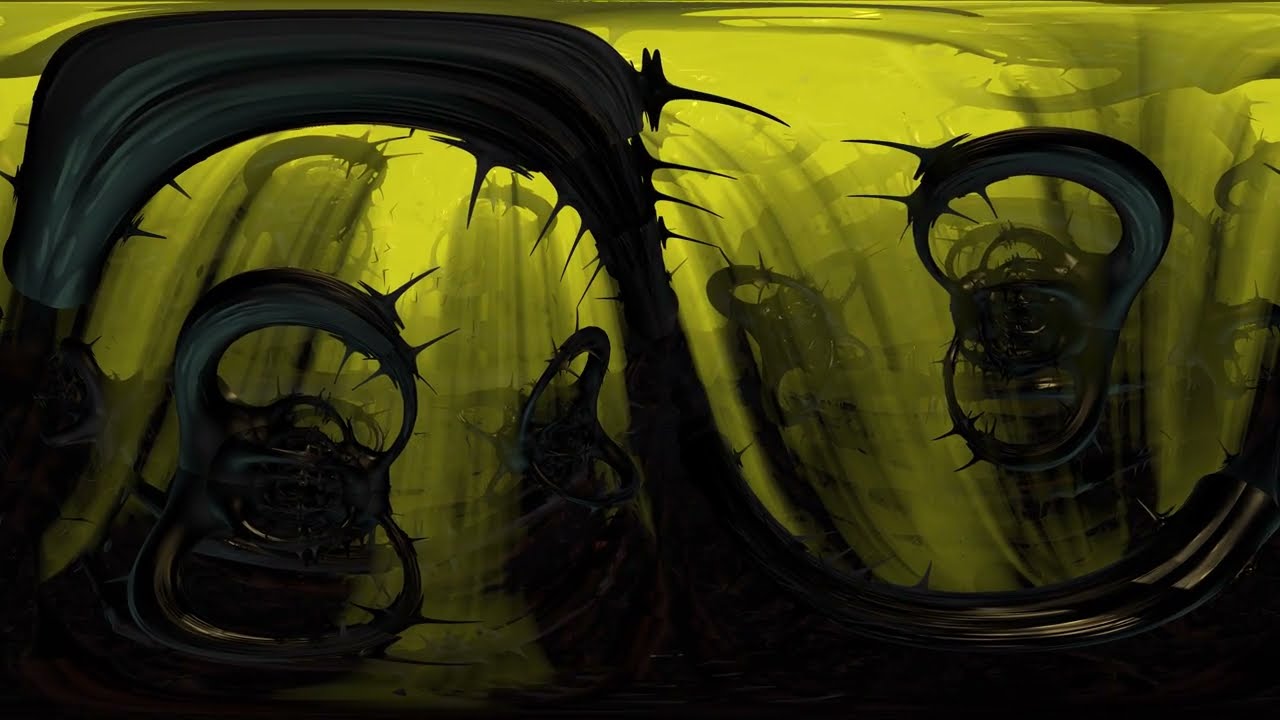The image depicts a surreal piece of artwork with a yellow background, featuring multiple ominous, black metal objects that have an oily sheen and are adorned with sharp, needle-like spikes. These objects are arranged in a spiraled, pointy design that seems to circulate, with their spiky tips prominently visible. There appear to be at least four of these menacing structures, though possibly more in the background, all set against the yellow backdrop. Some of the objects hint at a ride-like configuration with what seem to be alien-looking figures or faces peering out, which gives the scene an eerie, hellish atmosphere.